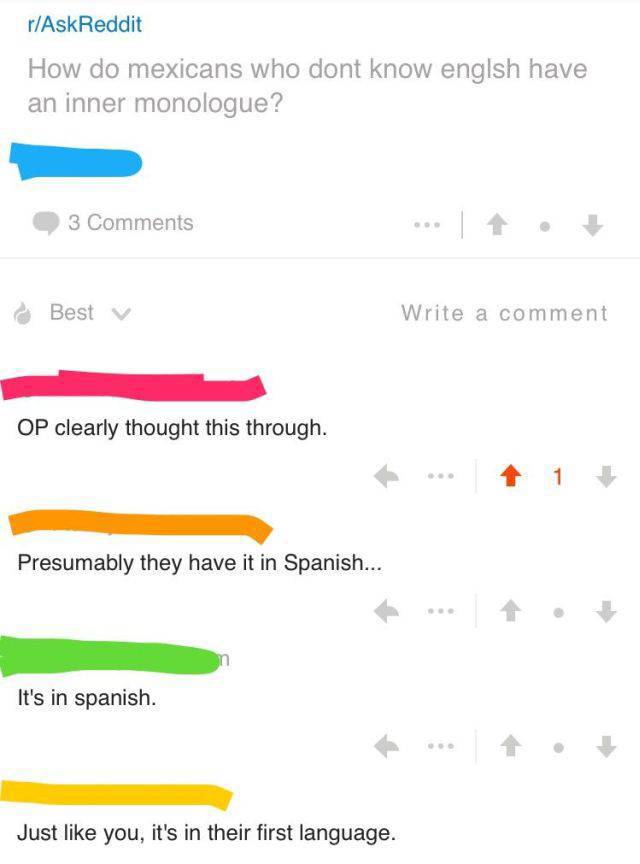The image features a screenshot of a Reddit thread from the subreddit r/AskReddit, displayed in the top left corner in teal-colored text with a capital 'A' and 'R'. Beneath the subreddit title, a gray text reads, "How do Mexicans who don't know English have an inner monologue?"

A thick blue line appears to have marked out a portion of the content below this line. In gray text, it displays "3 comments" followed by a long horizontal line. Further down, there's a red area that is also marked through, with the text "OP clearly thought this through" beside it. To the right, a red arrow pointing upwards indicates a single upvote.

Below these elements, a thick orange line is followed by the text "Underneath this, presumably they have it in Spanish..." Moving downward, another medium green line appears with the text, "It's in Spanish." Subsequently, a thick yellow line marks off another section where someone has commented, "Just like you, it's in their first language."

At the very top above the red line, the word "Best" is mentioned in gray, and about three inches to the right, also in gray, is the phrase "Write a comment."

Overall, the image is a detailed segment of a Reddit thread discussing the nature of inner monologues in different languages, specifically in the context of Spanish-speaking individuals.